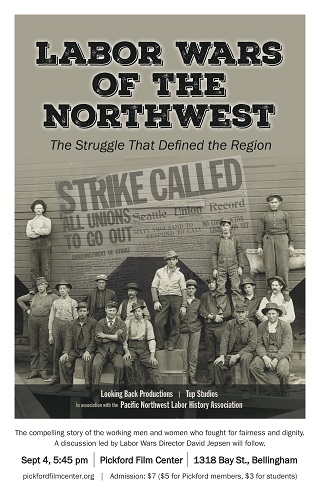A black-and-white poster titled "Labor Wars of the Northwest: The Struggle That Defined the Region" depicts a group of about 15 serious-looking Caucasian male workers from the early 1900s, suggesting they're on strike. The men, wearing various styles of hats, shirts, pants, suspenders, and jackets, are posed for a group photo. Overlaid on the image is text resembling a newspaper headline, "Strike Called, All Unions to Go Out," indicative of a historical labor strike. The production credits at the bottom read, "Looking Back Productions in association with Top Studios and the Pacific Northwest Labor History Association." Event details include a screening on September 4th at 5:45 p.m. at the Pickford Film Center, 1318 Bay Street, Bellingham, with an admission fee of $7, discounted rates for Pickford members and students, and additional information available at Pickfordcenter.org.